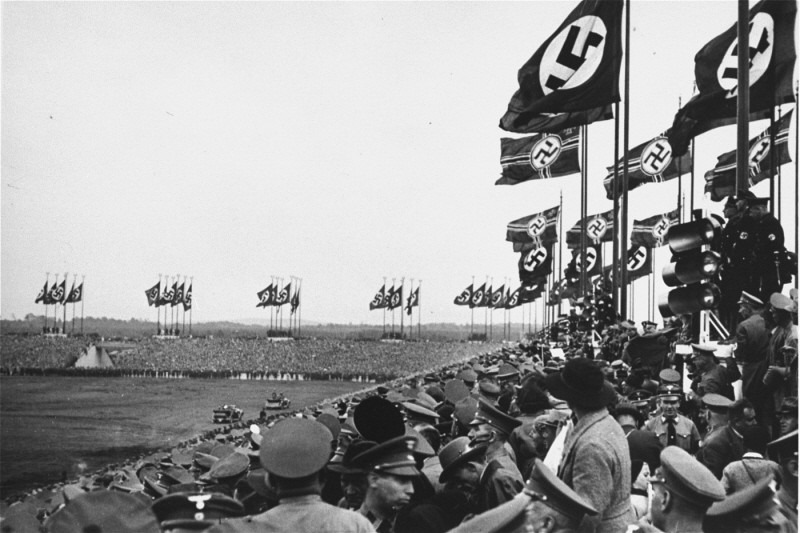This black and white photograph captures a grand Nazi parade in a large open amphitheater, most likely from the 1930s or early 1940s in Germany. The amphitheater is filled with thousands of spectators and military officials dressed in formal attire, including military caps and Nazi armbands. Women can be seen wearing tweed jackets and hats. The stands are adorned with at least 25 closely grouped Nazi flags, arranged in clusters of five on poles. The scene is further illuminated by large manned spotlights. On the flat field at the center, several military vehicles are visible, suggesting a military presentation or parade, possibly attended by high-ranking officials such as Hitler. The cloudy skies add a somber tone to this historical moment.